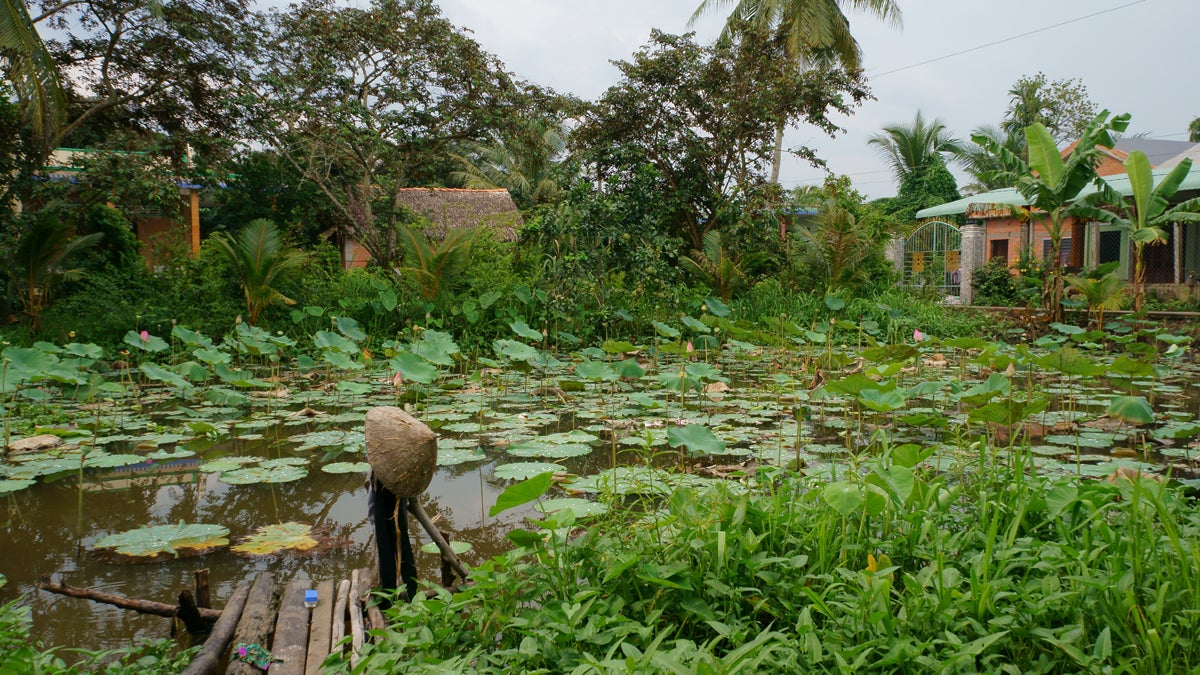The image depicts a serene outdoor setting of a tropical pond with prominent large lotus pads covering the water's surface, which is a murky brown. In the lower left corner of the pond, remnants of a small dock are visible, represented by old wooden slats. The pond is framed by taller grass with vibrant yellow flowers in the lower right corner and surrounded by various trees. A house with tropical palm and banana trees stands in the upper right corner. This dwelling features a blend of white and peach/orange hues and has an arched gate and a fence with yellow details in front. Adjacent to the pond, there are scattered bamboo poles and tree trunks on the ground. Amongst the foliage, a person is seen standing near the water, distinguished by a traditional Japanese bamboo umbrella and black pants, adding a cultural element to the scene.